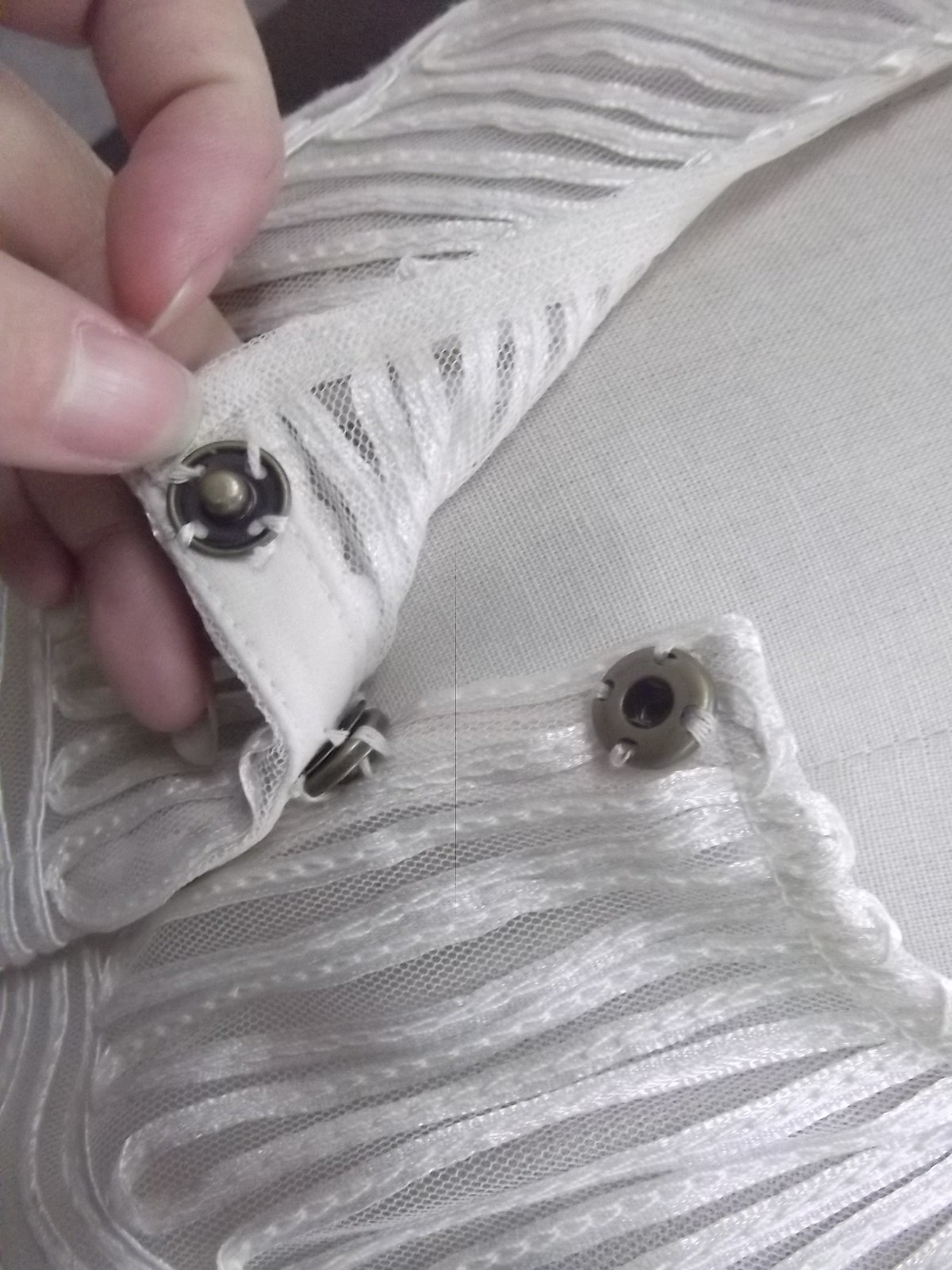This close-up image showcases a detailed view of a lacy white women's top. The fabric alternates between solid lacy white sections and sheer, net-like strips, creating a see-through effect. A hand with neatly manicured, unpainted long fingernails, presumably a white woman's, is pulling back at the collar area of the top to reveal two coppery brown snaps. The snaps are sewn securely, with visible stitching, and the top snap is undone, allowing a clear view of the fastening mechanism. The top appears to be displayed on a white, fabric-covered mannequin, suggesting this may be a design in progress or being presented for inspection. The setting of the image hints at an indoor environment, possibly within a home or a studio.